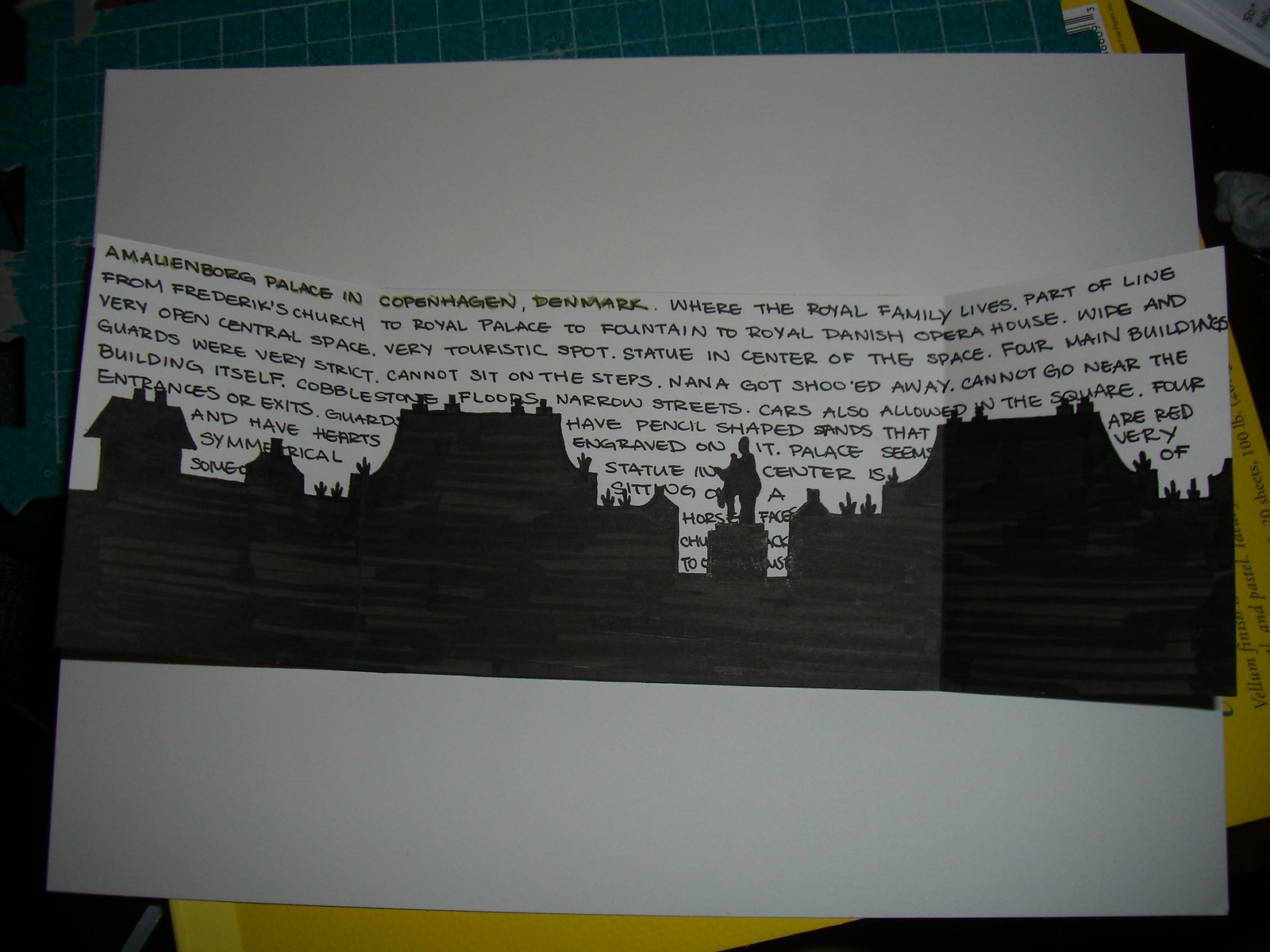The image depicts a detailed illustration on a cutout rectangular paper set against a larger blank white background. The paper, approximately occupying the middle third of the white sheet, features a blend of handwritten and printed text in shades of black and brown. The text reads, "Amalienborg Palace in Copenhagen, Denmark, where the royal family resides." This section also mentions the palace's location along a line from Frederick's Church to the Royal Danish Opera House, indicating significant touristic structures. Surrounding the text is an intricate black silhouette of the Amalienborg Palace buildings, complete with detailed rooftops, chimneys, and other architectural elements. Despite the predominance of white and black in the design, the background of the entire setup appears to have shades of green and yellow, adding a layer of depth and context to the depiction.